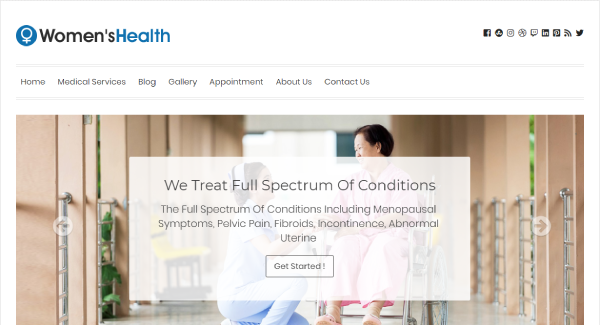Screenshot of the Women's Health Website

The screenshot captures the main page of the Women's Health website. Positioned at the top left of the screenshot is the Women's Health logo, with the word "Women's" in black and "Health" in blue. To the right of the logo are icons for social media platforms, including Facebook and Twitter, indicating that users can click on these icons to visit Women's Health's associated social media pages.

The website's navigation menu includes links to various sections such as Home, Medical Services, Blog, Gallery, Make an Appointment, About Us, and Contact Us. This menu suggests that users can explore a range of options including reading blog posts, viewing picture galleries, booking appointments, and learning more about the organization.

The central part of the screenshot features text highlighting that Women's Health treats a full spectrum of conditions. These conditions include menopausal symptoms, pelvic pain, fibroids, incontinence, and abnormal urine. There is a call-to-action button inviting users to get started.

In the background, a banner is partially visible, along with an image depicting a caring interaction between a nurse and a patient. The nurse is kneeling beside a wheelchair, speaking to an Asian woman who appears to be between 60 to 70 years old. The woman is smiling, creating a warm and compassionate scene. The setting suggests a rehab room equipped with support structures, indicating that it may be a space where patients with walking difficulties practice their mobility.

Overall, the screenshot conveys a comprehensive and supportive atmosphere, emphasizing the range of medical services offered by Women's Health.